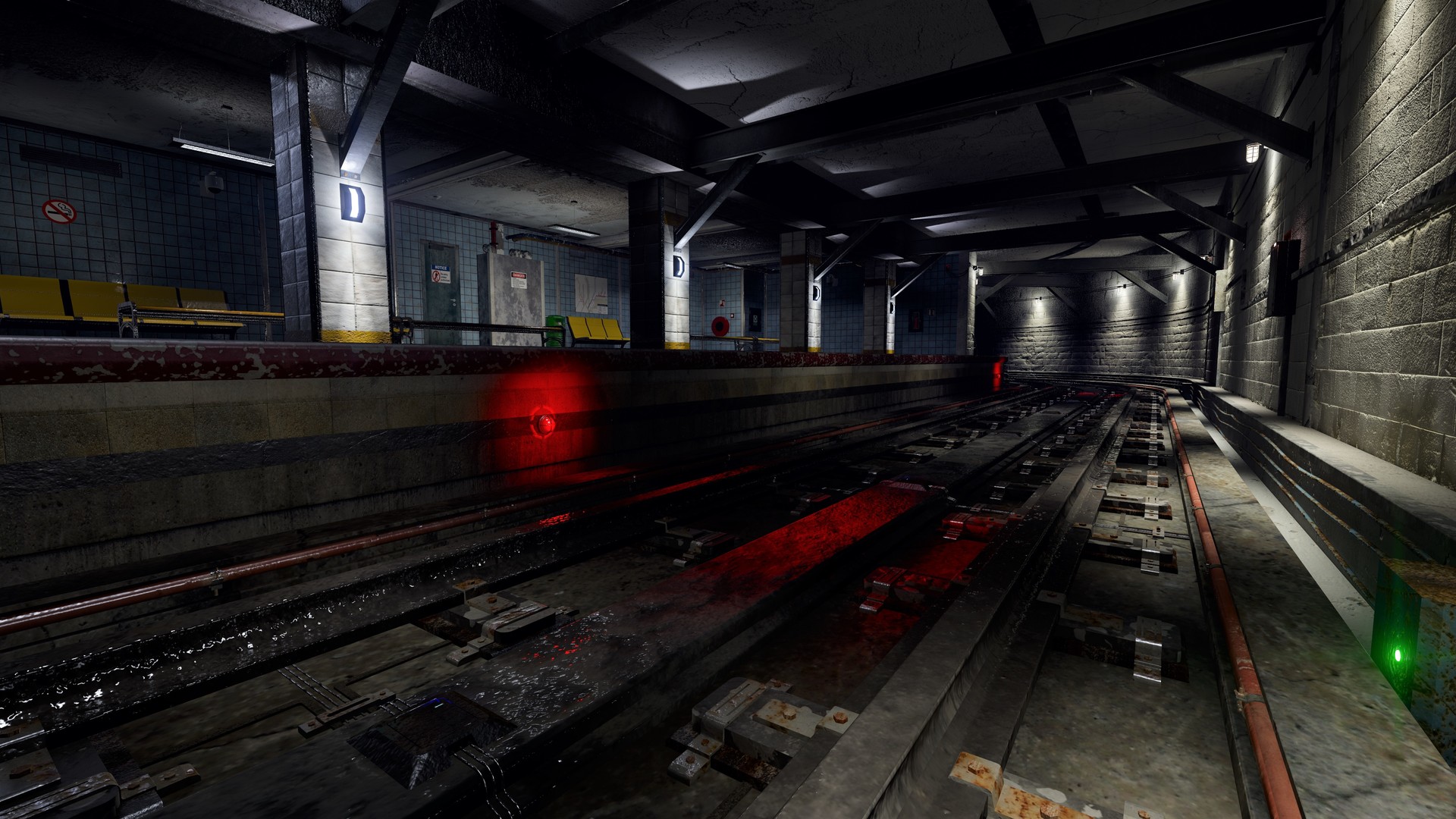This image depicts the dark interior of an underground subway station. The scene is centered around the black train tracks, which run diagonally upward from the lower left to the center of the picture. Illuminating the tracks are various lights, including a prominent red light reflecting onto the track and a green light in the lower right corner. On the left side, blue tiled walls and columns stretch along the platform, accompanied by a railing and some yellow seats. Contrast this with the right side, where gray brick-like tiled walls extend across and into the background. Despite the overall dimness of the station, there are lights that provide some illumination to the track and surrounding areas, suggestive of an eerie, videogame-like atmosphere. No people or vehicles are present, further emphasizing the station's desolate and immersive ambiance.